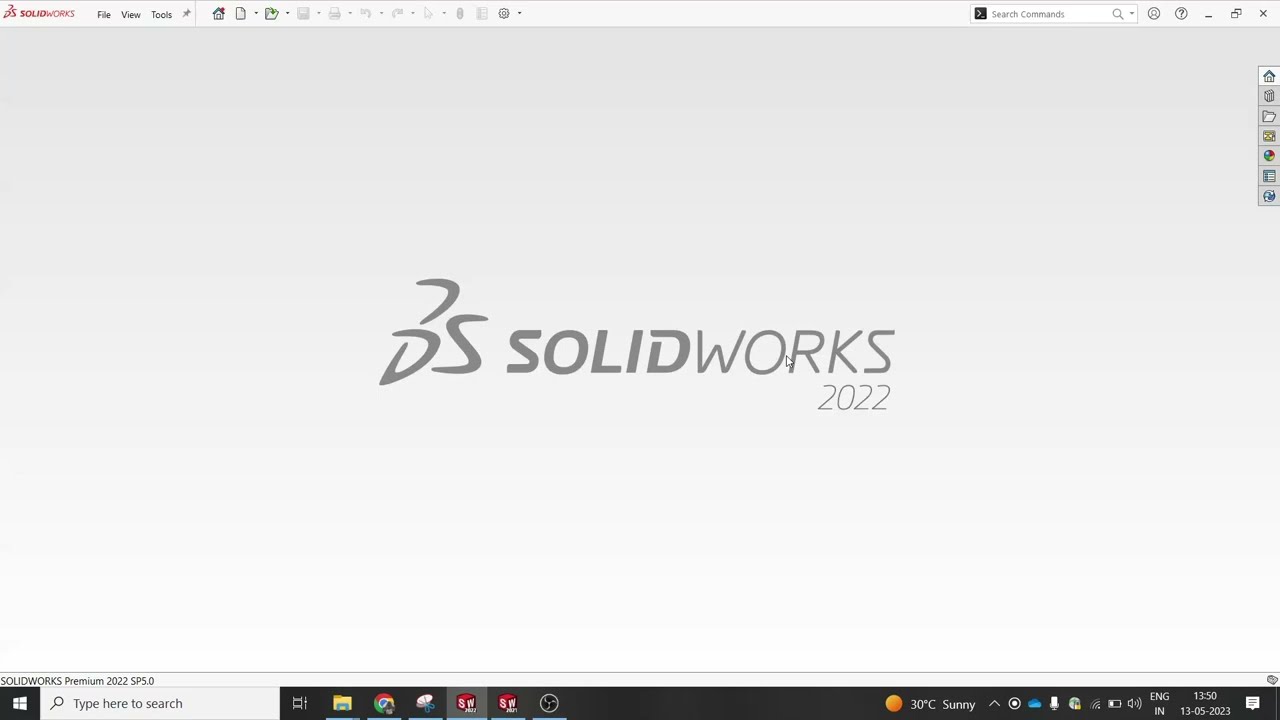This detailed screenshot captures a Windows computer screen showcasing the SolidWorks 2022 application. The top-left corner features a difficult-to-read red text, while adjacent to it, the toolbar displays options like File, View, and Tools. To the right, there's a search box. Dominating the center, the display exhibits the SolidWorks 2022 logo prominently in gray letters, with "BS" in bold and "SolidWorks 2022 SP5" beneath it in thinner font. A vertical toolbar on the right side contains various tool icons, though their specifics are unclear due to their distance and the low resolution of the image. Along the bottom, the black Windows taskbar hosts the Windows icon initiating the start menu, a search bar, and various other icons including Google Chrome and weather information. The background of the SolidWorks window transitions from white at the bottom to a light gray gradient towards the middle.